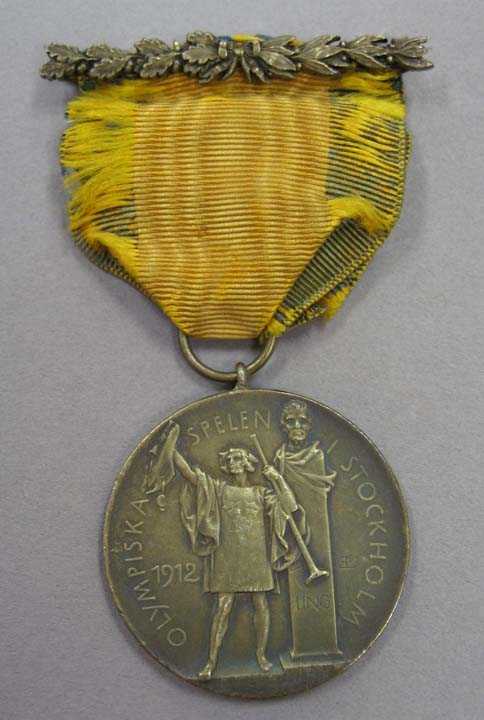This image showcases an antique Olympic medal from the 1912 Stockholm Games. The vertically aligned rectangular picture features the medal resting on a medium gray background. The medal is attached to a fabric ribbon which appears faded and slightly shredded along the edges. The ribbon, in a yellow tone, is adorned with an ornate metal filigree pin at the top, reminiscent of Greek cultural designs with intricate floral and vine patterns. 

At the bottom of the ribbon, a small metal hoop connects to a larger bronze-colored circular medal. The front of the medal depicts a Roman or Greek figure wearing a toga and holding a horn, with a statue and a pedestal beside him. The inscription reads "Olympiska Spelen" at the top, "Stockholm" to the right, and "1912" on the left. The detailed craftsmanship and tarnished color give it an authentically aged appearance, reflective of its historical significance as an Olympic award from over a century ago.